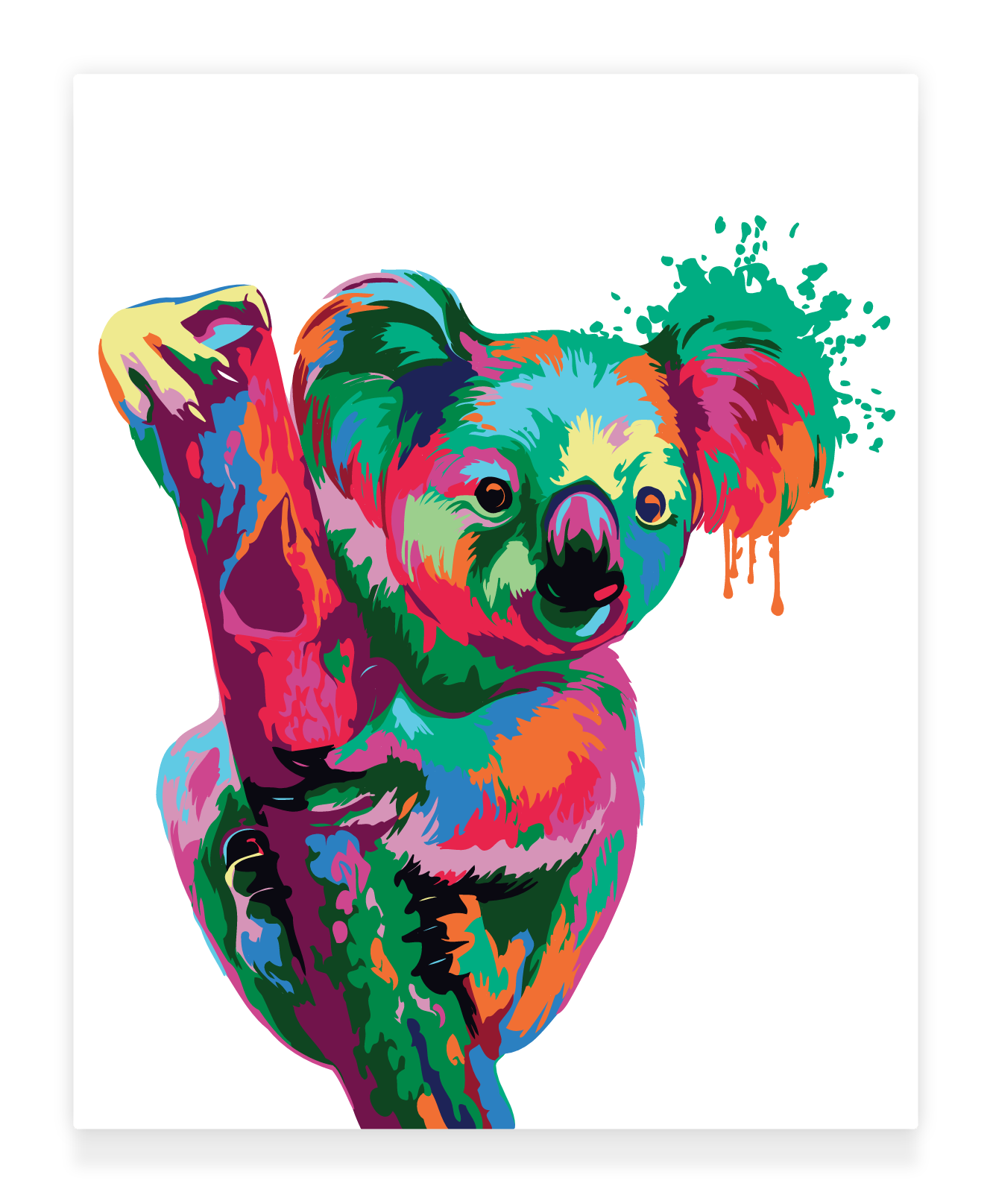This striking piece of art features a vividly colorful koala perched on a bamboo shoot, all set against a stark white background. The koala is painted in a dazzling array of colors, including shades of pink, orange, green, yellow, and blue, creating a mesmerizing spectacle. Notably, its left ear appears greenish, while the right ear resembles an ink splatter incorporating green and red hues. The koala's forehead is a blend of blue and green, with its purplish right side contrasting the greenish belly. One of its hands, distinctly yellow, is clasping the top of the bamboo, while the other hand grips the side, with its back legs similarly wrapped around the shoot. The bamboo itself is equally vibrant, showcasing a mix of purples, blues, oranges, pinks, and greens, adding to the image's dynamic and lively feel. The white background, capturing the art on what appears to be a rectangular surface, enhances the colorful koala's prominence, making it the focal point of the composition.